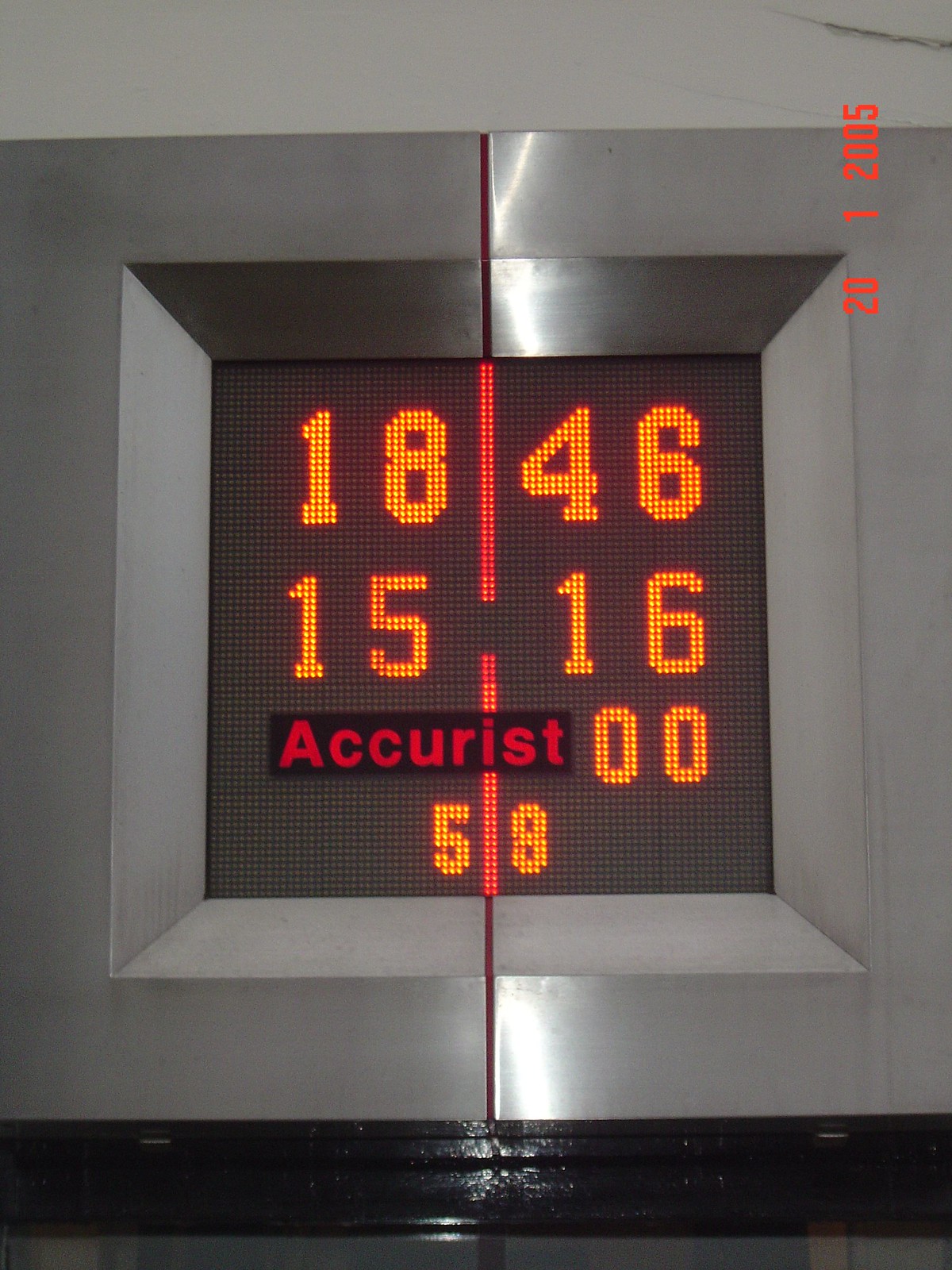This detailed image captures a digital display with a large-pixel, orange-colored readout. The numbers displayed are grouped and read as follows: "18" and "46" on the top row, "15" and "16" on the middle row, and "00" accompanied by "58" on the bottom row. The dark digital screen is encased within a recessed silver border. Distinguishing itself, the display features a red line running horizontally through its middle, which is separated in the center. Notably, the text "ACCURIST" is prominently shown on the left side of the "00," rendered in red font. The photograph also includes a date in the upper right corner that reads "20 1 2005," indicating that the photo might be relatively old, likely taken with an older camera. The lighting and reflections on the silver border suggest it was captured indoors.